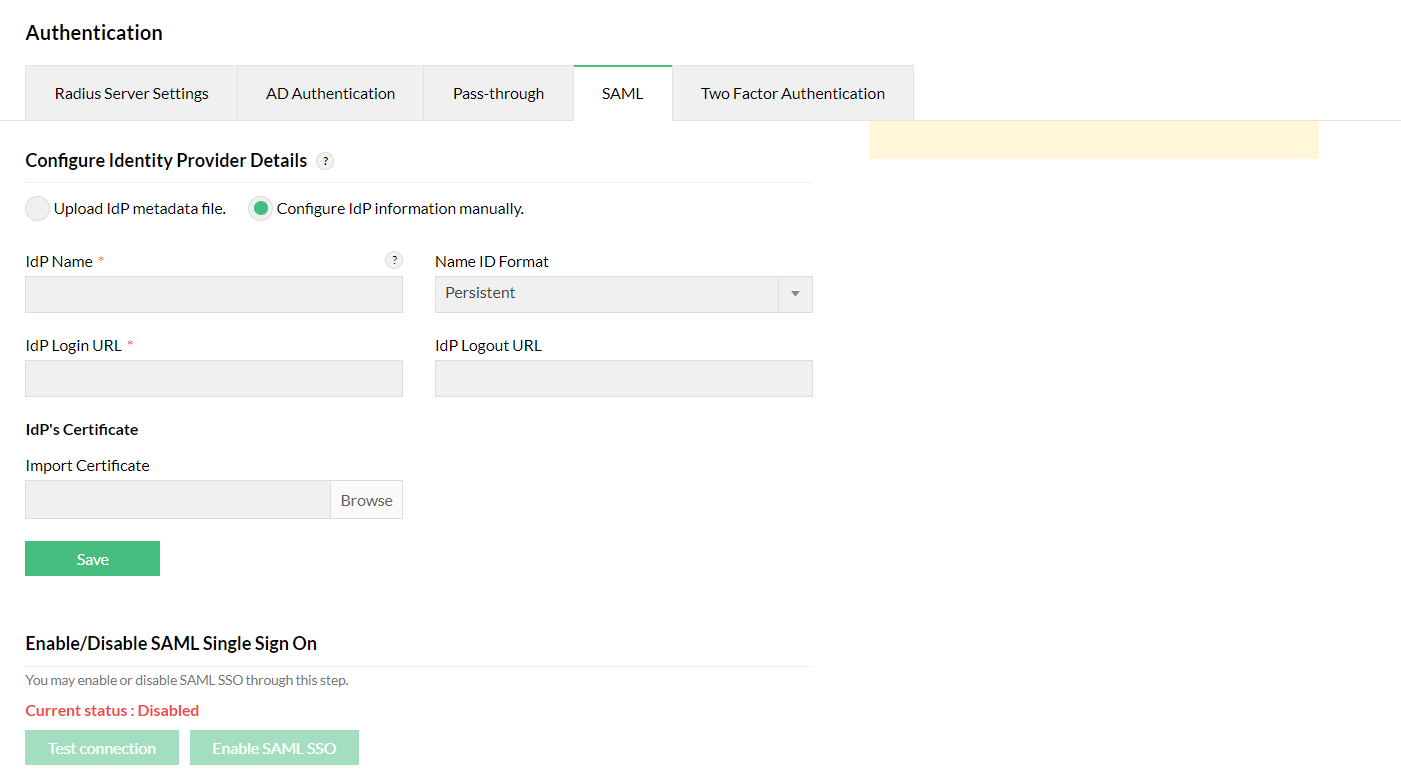**Detailed Caption:**

The image displays a user interface for configuring various authentication methods on a system. At the top, the following authentication options are listed: "Admin Authentication", "RADIUS", "Server Settings", "AD Authentication", "Pass-Thru", and "Two-Factor Authentication". Among these options, "SAML" is highlighted, indicating it is the currently selected method.

Below the highlighted "SAML" option, there is a detailed configuration section titled "Configure Identity Provider Details". This section provides options to either "Upload IDP Metadata Files" or "Configure IDP Information Manually".

For manual configuration, the following fields are available:
- "IDP Name"
- "Name ID Format"
- "Persistence"
- "IDP Login URL"
- "IDP Logout URL"
- "IDP Certificate", with an option to "Import Certificate" through a "Browse" button.

At the bottom of this section, there is a "Save" button and a toggle option labeled "Enable/Disable SAML Single Sign-On". A note under this option explains that you may enable or disable SAML Single Sign-On (SSO) through this step. 

The current status of SAML SSO is indicated as "Disabled".

Lastly, there are repeated lines indicating the connection settings: "Connection, Enable SAML SSO", emphasizing the functionality to enable SAML Single Sign-On in the system’s connection settings.